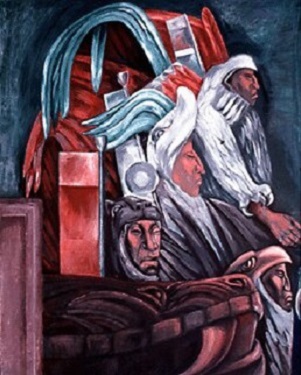The painting portrays a dynamic and intricate scene with a dark blue-gray background, featuring multiple figures adorned in ceremonial garb. The foreground highlights a squatting man dressed in a brown robe. His pose draws attention to another figure in front of him, whose head and shoulder are visible. Above this pair, a larger figure appears, bearing an elaborate headdress that resembles a bird—possibly an eagle or another avian creature—crafted with white and transitioning to gray feathers. This headdress seems to be part of a larger, intricate costume that may include elements resembling armor or ceremonial suits.

The composition suggests a tiered arrangement, with other figures aligned behind and above, their faces emerging somewhat flatly from the background. Each of these figures wears distinct headdresses, one possibly shaped like a dolphin and another like a lion, adding to the scene's ethereal and mysterious quality. The men seem to be facing the right, their arrangement suggesting movement or a hierarchical structure.

In the background, shades of dark teal or blue-gray add depth and contrast, while streaks of red or blue flow behind the figures, enhancing the surreal atmosphere. A reddish-brown object, possibly a barrel or a box, sits to the left, adding to the composition's complexity. Overall, the painting's rich details and vibrant colors create a captivating and enigmatic tableau, blending cultural elements with a sense of mythical narrative.